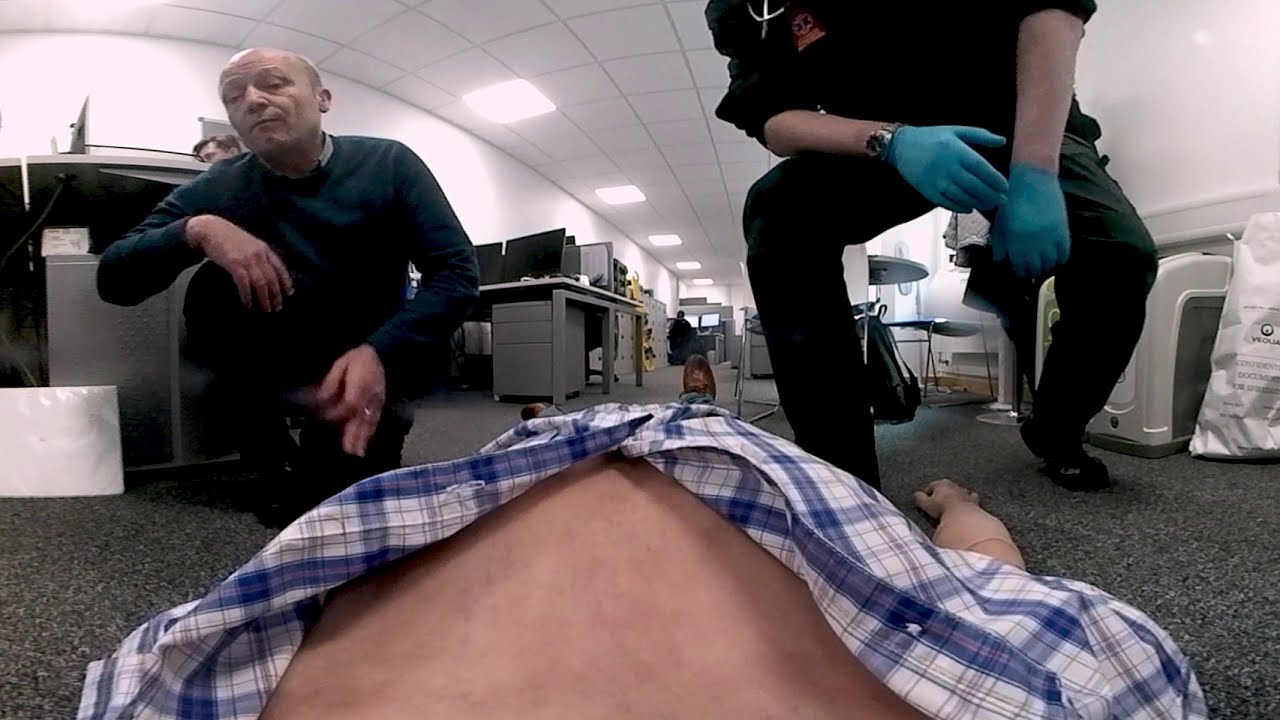The image is an interior color photograph taken from the perspective of a man lying on a speckled black floor or rug in an office setting. The man, who has fair skin, is wearing a partially unbuttoned blue and white plaid shirt, revealing part of his chest, and brown shoes. Surrounding him are concerned individuals. To his left, an older man in a dark green sweater over a collared shirt is kneeling and looking down with concern. On the right, a person in dark green scrubs is kneeling down with turquoise gloves and a watch, seemingly an EMT or medical professional. This person appears to have a stethoscope around their neck. In the background, gray desks equipped with computers and monitors are visible, adding to the office environment. The ceiling features white grid-style tiles with rows of lights, completing the scene of a medical emergency in a professional setting.